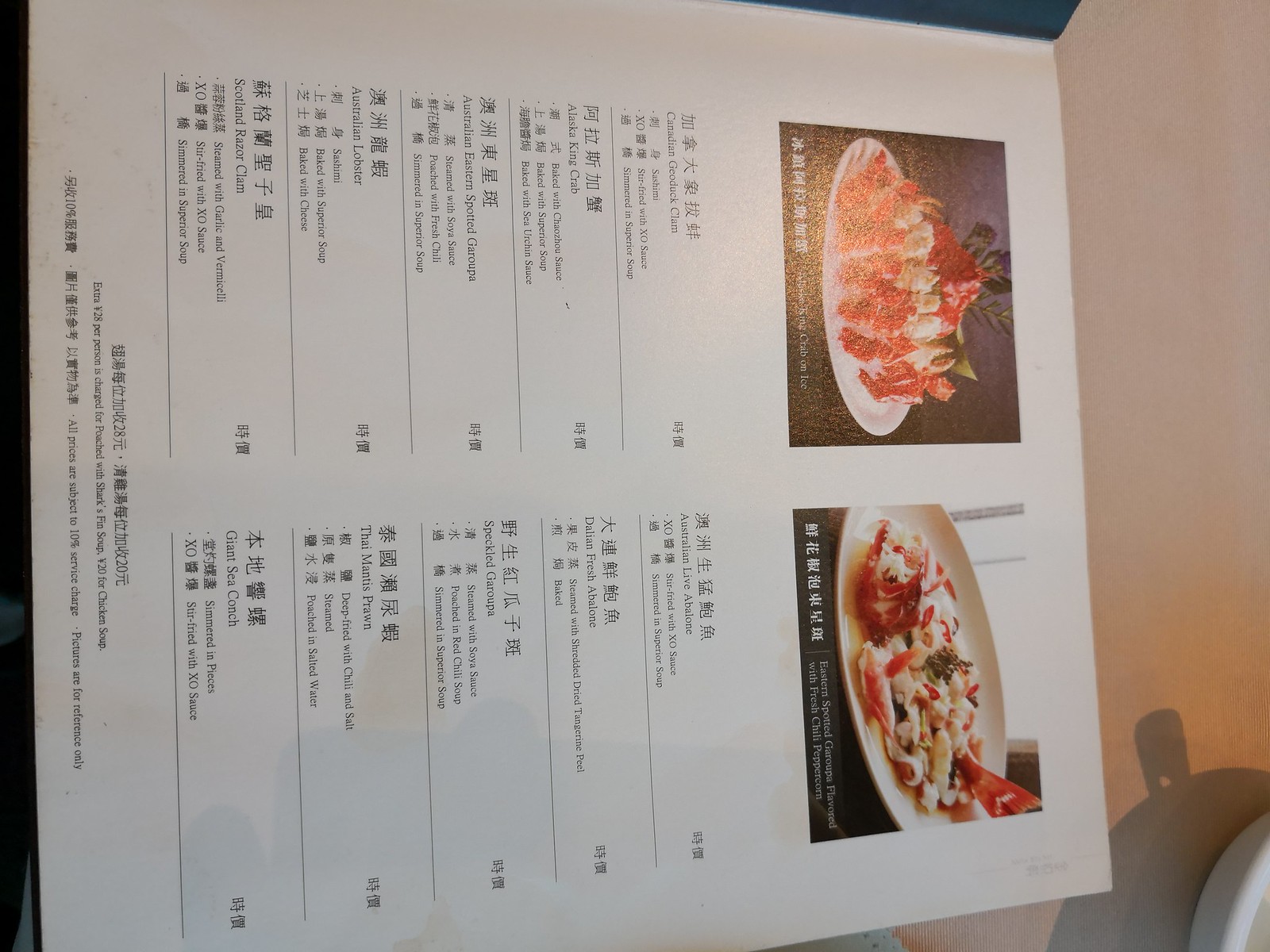The photograph captures a menu set sideways on a light, clear table. In the upper right-hand corner of the image, a white ceramic object, possibly a saucer, is visible, accompanied by its shadow which reveals a small handle. The menu itself features two primary images at the top. The image on the left displays an assortment of food items arranged on a white plate against a black background. The image on the right showcases a smaller spread of food on a cream-colored dish with a window serving as the backdrop.

Beneath these images, the menu is divided into two columns. Each column aligns with the corresponding image above, listing descriptions of the dishes on the left and their prices on the right. Unfortunately, the text is either too blurry to discern or written in an Asian language. At the bottom of the menu, there is an explanatory section, presumably offering further details about the items or the dining experience, all in Asian lettering. This section is bordered by a thick black stripe running across the lower edge of the menu.